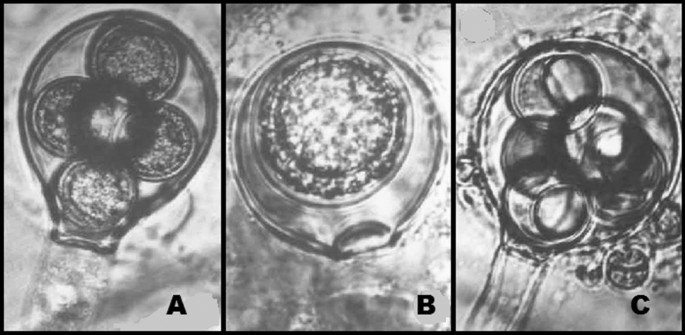The image is a horizontally rectangular black-and-white composition featuring three vertically rectangular frames labeled A, B, and C, highlighted with thin black borders separating each frame. Each frame seems to depict a microscopic view of potentially biological significance, possibly cellular organisms or early-stage embryos.

Frame A resembles the shape of a light bulb and contains multiple overlapping circular structures. Four of these circles converge at the center, encompassed by a larger black circle set against a gray background. 

Frame B features a single central circle resembling a textured diamond set within a ring, possibly representing a different stage or a distinct organism.

Frame C mirrors the formation in A but appears rounder with a denser cluster of smaller overlapping circles within the encompassing membrane. 

All three frames, entirely devoid of color, illustrate a progression of growth or developmental stages of a microscopic subject, with labels A, B, and C providing the only textual context.